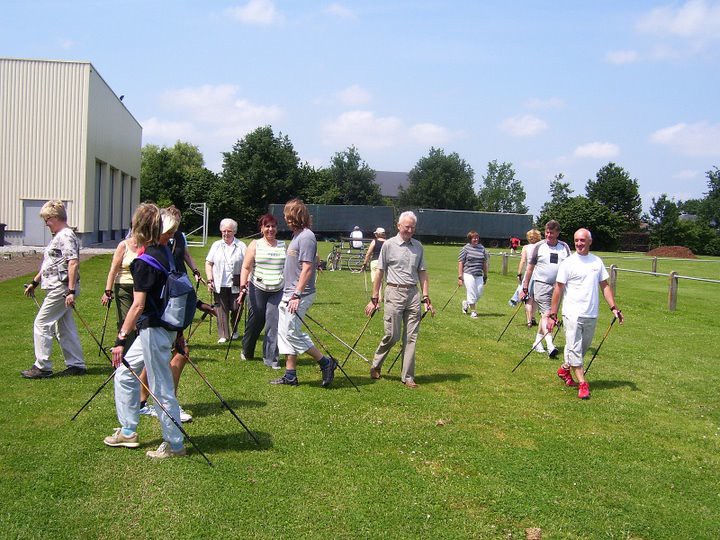The photograph captures a vibrant outdoor scene featuring a diverse group of approximately a dozen individuals, predominantly senior citizens estimated to be over the age of 55, walking across a well-trimmed, lush green field. They are using trekking poles, characterized by loops at the handles for stability and to reduce strain on their legs—a common aid for hikers. These poles appear to be attached to the walkers' wrists, adding to the supportive function. The individuals are dressed in a mix of loose, casual clothing, including t-shirts, polo shirts, and shorts, reflecting a relaxed atmosphere.

In the background, a gray industrial-style building stands to the left, suggesting the field could be part of a larger sports or recreational area. Further back, within the expansive setting, there is a running track encircled by a rail, soccer goals, and small bleachers, emphasizing the multifunctionality of the space. The backdrop also features towering, vibrant green trees and a light blue sky dotted with a few scattered clouds, completing the serene outdoor environment.